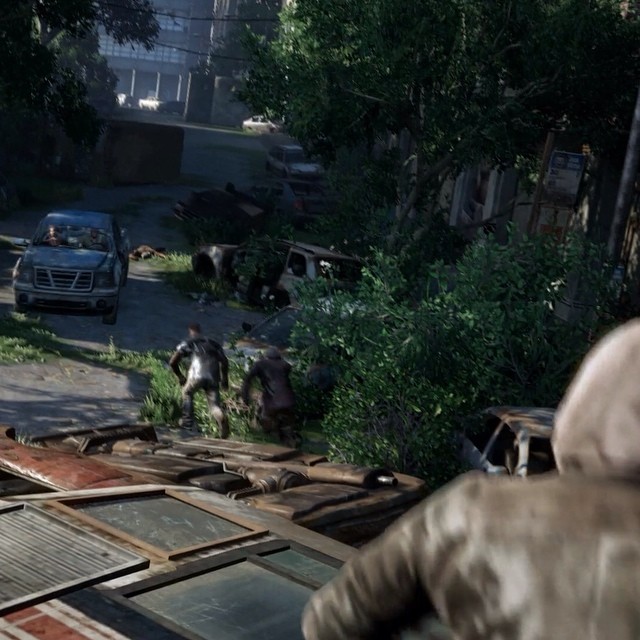The image is a screen capture from a video game, depicting a tense and chaotic scene. The main character, seen from behind and over the shoulder, is wearing a brown leather jacket with the hood up, partially obscuring his head from the left side. He appears to be either crouching or standing atop a makeshift structure composed of various panels, giving the impression of a rooftop or junk pile. His position is slightly blurred, adding a dynamic feel to his vigil.

In the foreground, the character is observing a scene below, where several wrecked cars are scattered, including one overturned vehicle. Behind this car, two men are cautiously sneaking forward, adding a layer of suspense as they converge towards the center of the image. Surrounding the area is dense foliage, which blends into a rough, unpaved driveway extending into the background. A blue car is visible in the distance, traveling along this rugged path towards the viewer. The driver of the approaching car can be seen through the windshield, further heightening the anticipation of what might unfold next.